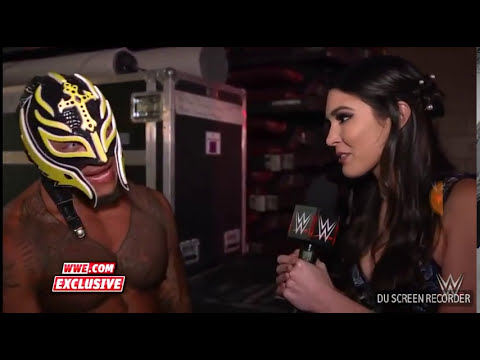This is a detailed screenshot taken from a backstage interview for WWE, featuring the wrestler Rey Mysterio and a young brunette interviewer. The photo captures them from the waist up, with Rey Mysterio on the left, shirtless and adorned with intricate chest tattoos. His iconic black and yellow luchador mask features a distinctive cross on the forehead and elaborate yellow highlights around the eyes and cheeks. On the right, the female interviewer has long dark hair and dark eyeliner, and she is holding a WWE-branded microphone.

In the background, there are large, gray equipment crates, indicating a behind-the-scenes setting. Text overlays on the image reveal additional context: "WWE.com Exclusive" is displayed on the wrestler's chest, while "DU Screen Recorder" is noted at the bottom right corner. To the right, beneath the interviewer, the WWE logo is also visible, adding to the authenticity of the scene.